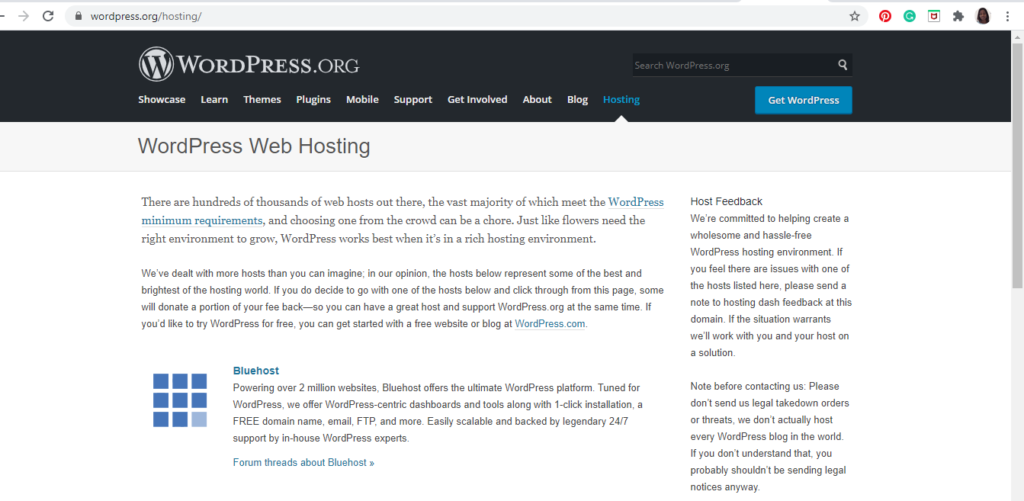**Detailed Caption:**

The webpage falls under the category of websites and features the URL "wordpress.org/hosting". At the top of the page, there is a search bar with a star icon within it, allowing users to bookmark the page. To the right of the search bar is the Pinterest logo. Additionally, there is a green circle containing a 'C', along with several other icons: a puzzle piece, a profile picture, and another icon.

Directly below these elements, the top navigation bar of the page is rendered in black and displays "wordpress.org". This bar includes a search engine for quick access to content. Below this black bar is a white menu that lists various sections such as Showcase, Learn, Themes, Plugins, Mobile, Support, Get Involved, About, Blog, and Hosting. The "Hosting" section is highlighted in blue letters.

Adjacent to this menu, there is a prominent blue box labeled "Get WordPress". Underneath this box is a gray bar with the text "WordPress Web Hosting". Following this, the main content area comprises several paragraphs discussing web hosting, though the text is extremely small.

At the bottom of the main content, there is a reference to "Bluehost," accompanied by a grid of nine squares. Eight of these squares are dark blue, while the one in the lower right corner is gray. This visual element likely represents a form of branding or a graphical indicator related to Bluehost services.